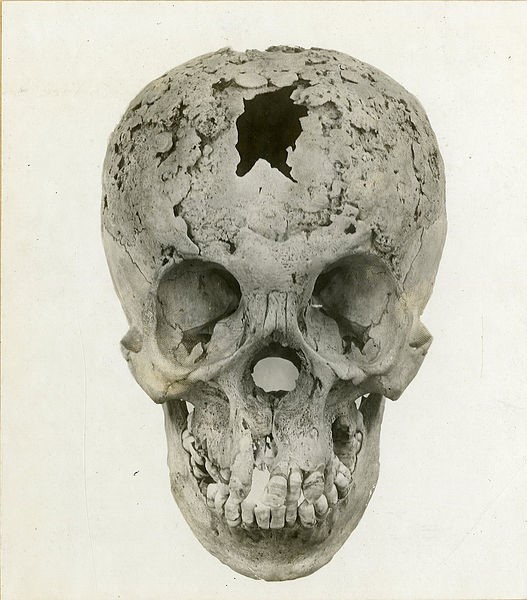The image depicts an ancient human skull, set against an off-white background, and seemingly taken in black and white. The skull shows significant wear and damage, particularly with a prominent gaping hole at the top of the head, suggesting a fatal blow. The bone around the hole appears chipped and flaked. Large eye sockets stare blankly, and the nose is completely missing, leaving a see-through cavity. The mouth is slightly deformed, with most of its teeth still intact, although one front tooth and several upper teeth on the left side are missing. The interior of the skull is notably black in color, visible through the damaged areas. The overall gray hue of the skull, coupled with its deteriorated condition, hints at its probable ancient origins, possibly unearthed during an archaeological dig.